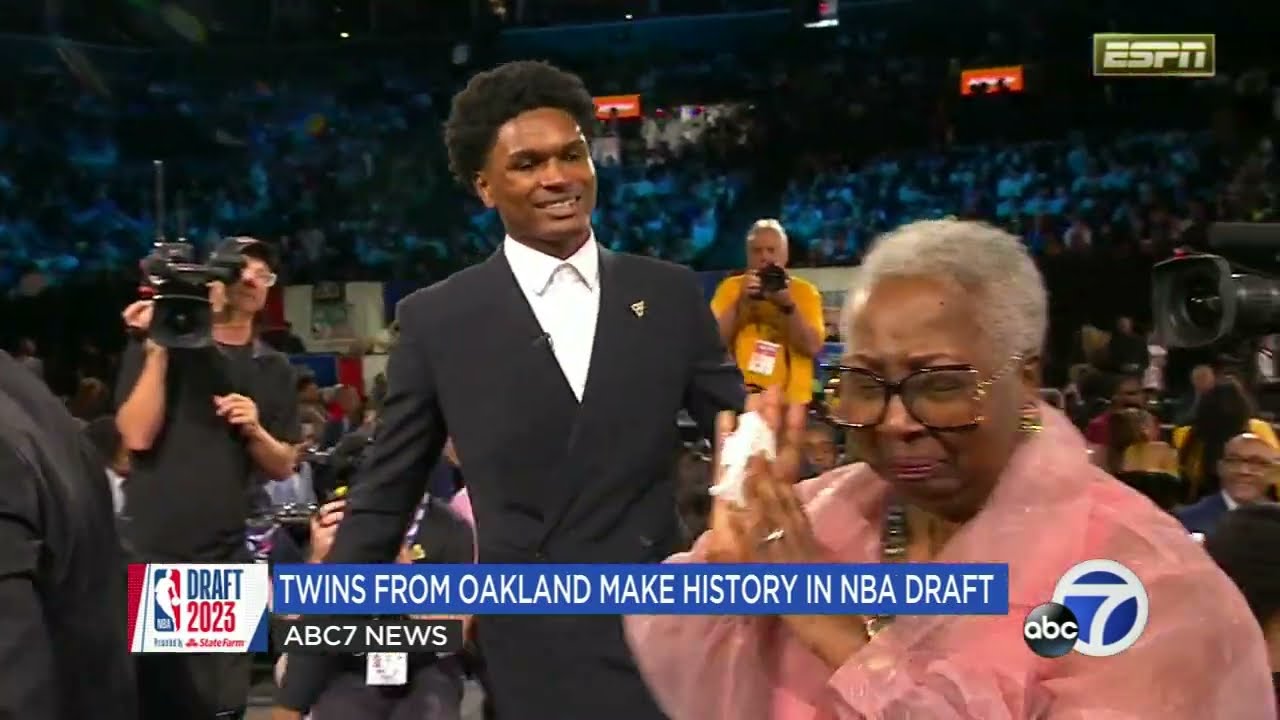In this image, we see a lively and emotional moment captured during ABC7’s coverage of the NBA Draft 2023, presented by State Farm. The headline reads, "Twins from Oakland make history in NBA Draft," alongside the ABC7 News and NBA Draft 2023 logos. In the foreground stands an African American man, tall with a dark complexion, wearing a sophisticated black suit, a white dress shirt, and a pin on his lapel. His confident smile reveals his teeth, and his dark, mini afro frames his face as he looks affectionately down at an African American woman to his right. 

This woman, presumably his mother, wears a vivid pink outfit with a translucent quality and large, purple-rimmed glasses. Her short gray hair complements her noticeable gold earrings. Her expressive face shows a mixture of pride and happy tears, as she clasps a cloth in her hands, held close in front of her chest. Surrounding them is a bustling scene; photographers and videographers with cameras capture the historic and celebratory atmosphere. Notably, one man in a dark yellow shirt holds a black camera above his head, while another, wearing a black t-shirt and hat, stands to the left aiming his camera.

In the background, a stadium crowd, seated in bleachers and on the court, adds to the excitement, with a prominent ESPN banner with a green background in the upper-right corner of the image. The entire scene exudes a sense of achievement and joy.